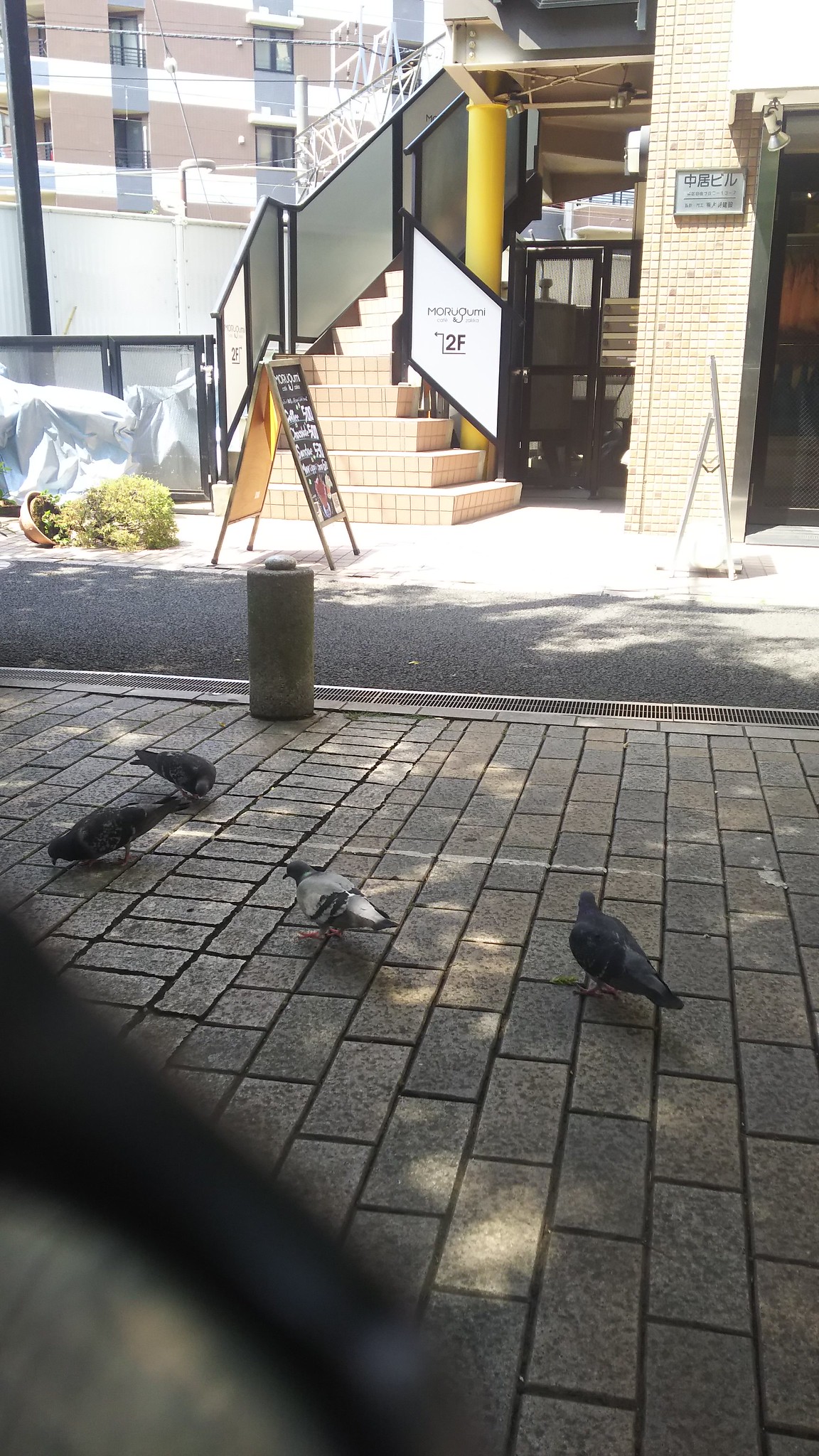This image captures a serene urban street scene, likely in an Asian city, characterized by its cleanliness and attention to detail. A yellow brick building stands prominently, adorned with a sign featuring Asian characters, possibly kanji. Access to this building is provided via a staircase made of pale yellow tiles, accompanied by a black iron railing with frosted glass panels. Adjacent to the stairs is a yellow-painted column. In the background, another tan-colored building features black-framed windows and wrought iron balconies.

The sidewalk in the foreground is meticulously paved and populated by four pigeons pecking around. Drain covers are evident, ensuring proper drainage in the area. Amongst the street furniture is a small pedestal near a drain on the border between the sidewalk and the asphalt street. A potted, fern-like plant lies toppled over, possibly due to wind, waiting to be righted by a passerby. Close to the steps of the yellow brick building is a sign that resembles a lunch menu chalkboard, indicating the presence of a nearby restaurant. This well-maintained scene showcases a blend of urban structures and subtle natural elements.